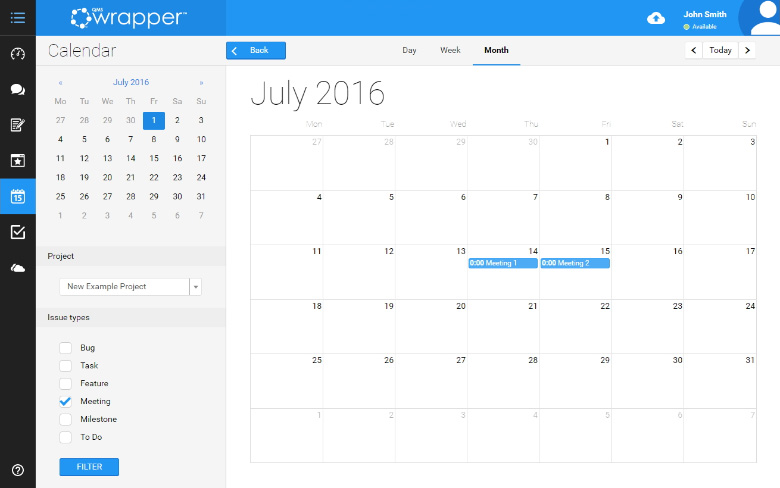This screenshot captures a detailed view of a comprehensive calendar application interface. At the top, there's a blue navigation bar. On the left side of this bar, "Wrapper" is displayed in white text beside a Pentagon logo. On the right side, the bar features a blue cloud icon with an arrow, indicating synchronization or upload functionality. Next to this icon, the user name "John Smith" is displayed in white, along with their status denoted as "Available."

On the left side of the screen, a black vertical sidebar houses a series of eight icons. From top to bottom, these icons are: a menu button, settings, chat, notes, a square with a star, calendar (highlighted in blue to show the active section), a box with a checkmark, and another cloud icon. At the very bottom of the sidebar, there is an additional question mark icon, likely for help or more information.

To the right of the sidebar, the main calendar section is displayed with a gray vertical sidebar. This secondary sidebar includes a labeled section for projects. Within this section, a dropdown menu shows "New Example Project." Below, there is a subsection for "Issue Types" featuring a list of checkboxes for different issue categories that can presumably be included or excluded in the calendar view.

This detailed interface layout suggests a robust, user-centric design aimed at facilitating project management and scheduling tasks efficiently.